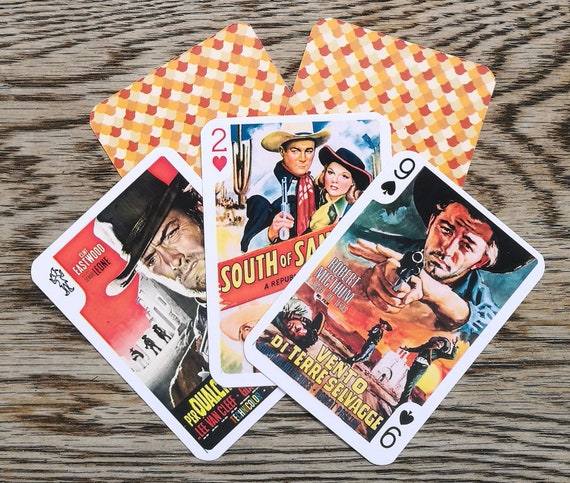The image shows five playing cards laid out on a distressed wooden surface. Three cards are face up, while two are face down featuring a checkered pattern in red, white, and orange. The face-up cards depict characters from Western movies. The nine of spades showcases Robert Mitchum in a dramatic pose, holding a gun with one hand and pulling the trigger with the other, connected to the title "Vento di Terra Selvagi". The two of hearts features a man and a woman in cowboy hats, labeled "South of Something," with the man wielding a pistol. The third card appears to be a joker, displaying an image of Clint Eastwood. The wooden background and the detailed illustrations on the cards strongly evoke a classic, rugged Western theme.